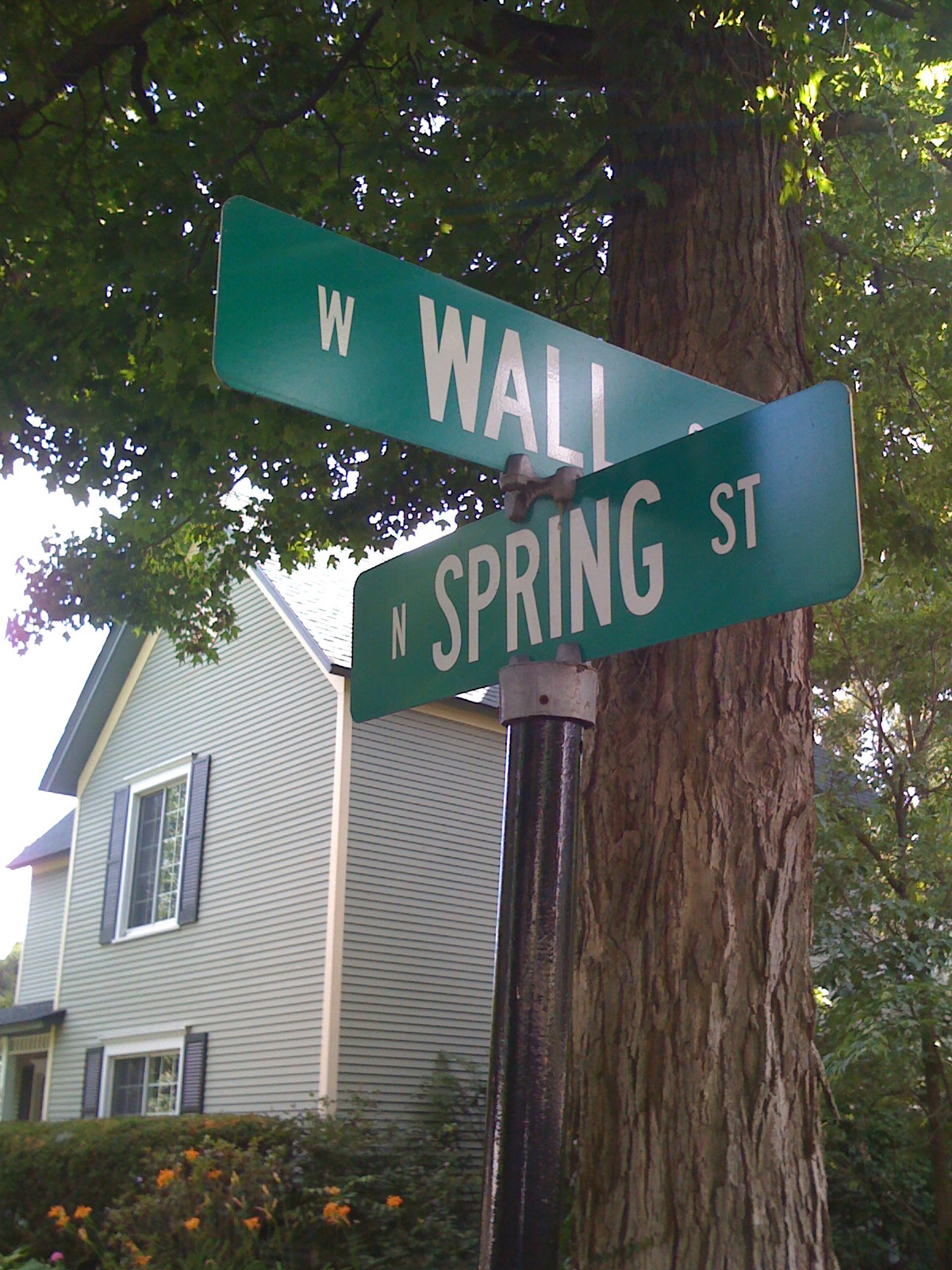The photograph captures a detailed view of a street intersection, specifically where North Spring Street and West Wall Street meet. The street signs, which are arranged in a criss-cross fashion similar to propeller blades, have a green solid background with bold white lettering. They are mounted on a silver metallic pole. Adjacent to the pole on the right is a tall and straight tree, featuring a thick barky trunk and lush green leaves extending to the top. To the left of the signs stands a two-story house clad in light blue vinyl panels with white trim edges. The house has two windows on the left side with white borders and bluish shutters. The roof of the house appears to be a darker blue shade. In the lower left-hand corner of the image, a bush with orange flowers is visible, which is fenced around the house. The sky appears white due to the lighting, indicating a sunny day.